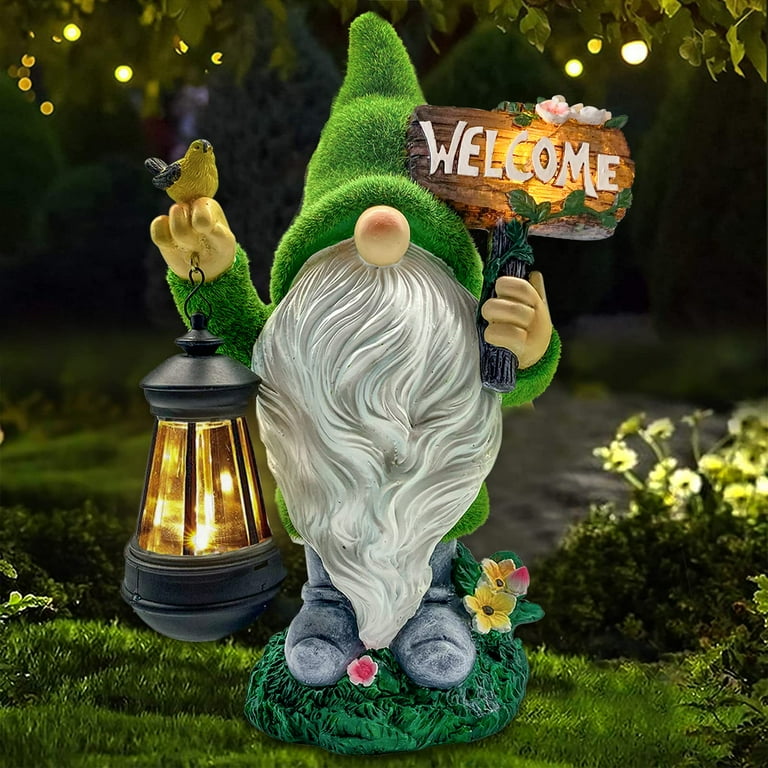This digital artwork depicts an enchanting nighttime scene featuring a whimsical garden gnome nestled in a lawn. The gnome, positioned centrally in the image, sports a green fuzzy hat pulled down over his eyes, revealing only his slightly upturned, light brown nose beneath. He proudly displays a long, flowing white beard that cascades down to his feet, covering his entire torso. His feet are adorned with gray boots, standing firmly on a patch of dark green grass.

In his right hand, he raises a black lantern emitting a soft glow, which illuminates the nearby area. A yellow bird with black wings and a tail perches delicately on his hand. His left hand, lifted near his head, holds a rustic sign made from a tree stick, bearing the word "welcome" in white letters on a wooden plaque. This sign is decorated with green vines and pink flowers, adding a charming touch to the gnome's appearance.

Surrounding the gnome are small bursts of color from yellow and pink flowers, integrated seamlessly with the green grass. The background features hints of trees and foliage, with the night sky softly illuminated by six small lights shining through the tree line on the right side of the image. A few leaves hang down from the top, adding depth and a serene, natural ambiance to this delightful scene.